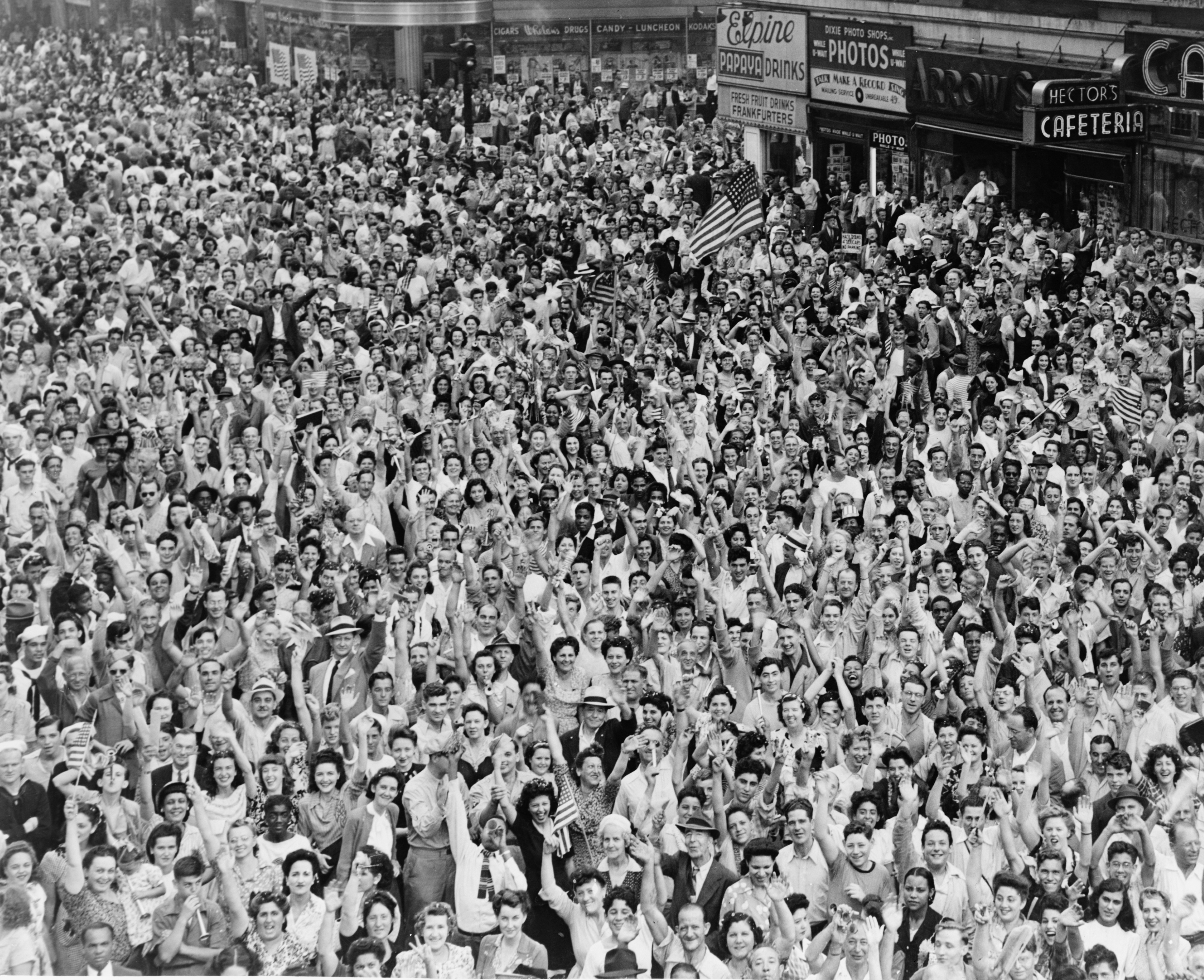A black and white aerial photograph shows a large crowd of people, with the forefront of the crowd facing the camera. The photograph captures the scene from an angled top-down perspective. In the background, specifically the upper left-hand side of the image, people appear to be facing away from the camera. The image exudes an older, historical ambiance, which is particularly highlighted by the signages and storefronts visible in the shot.

On the upper right-hand side, several signs adorn what looks like a metal storefront. Among them are distinct signs for Hector's Cafeteria, photo services, an arrow sign pointing towards a direction, and an Alpine drink advertisement. These signs indicate various small shops housed within a singular building. 

Adjacent to this building is a road, and beyond that, another store emerges into view from the upper center of the frame. This appears to be a candy store, adding to the quaint, nostalgic feel of the scene. The composition of the image, with its densely packed crowd and identifiable period storefronts, offers a vivid glimpse into a bygone era.